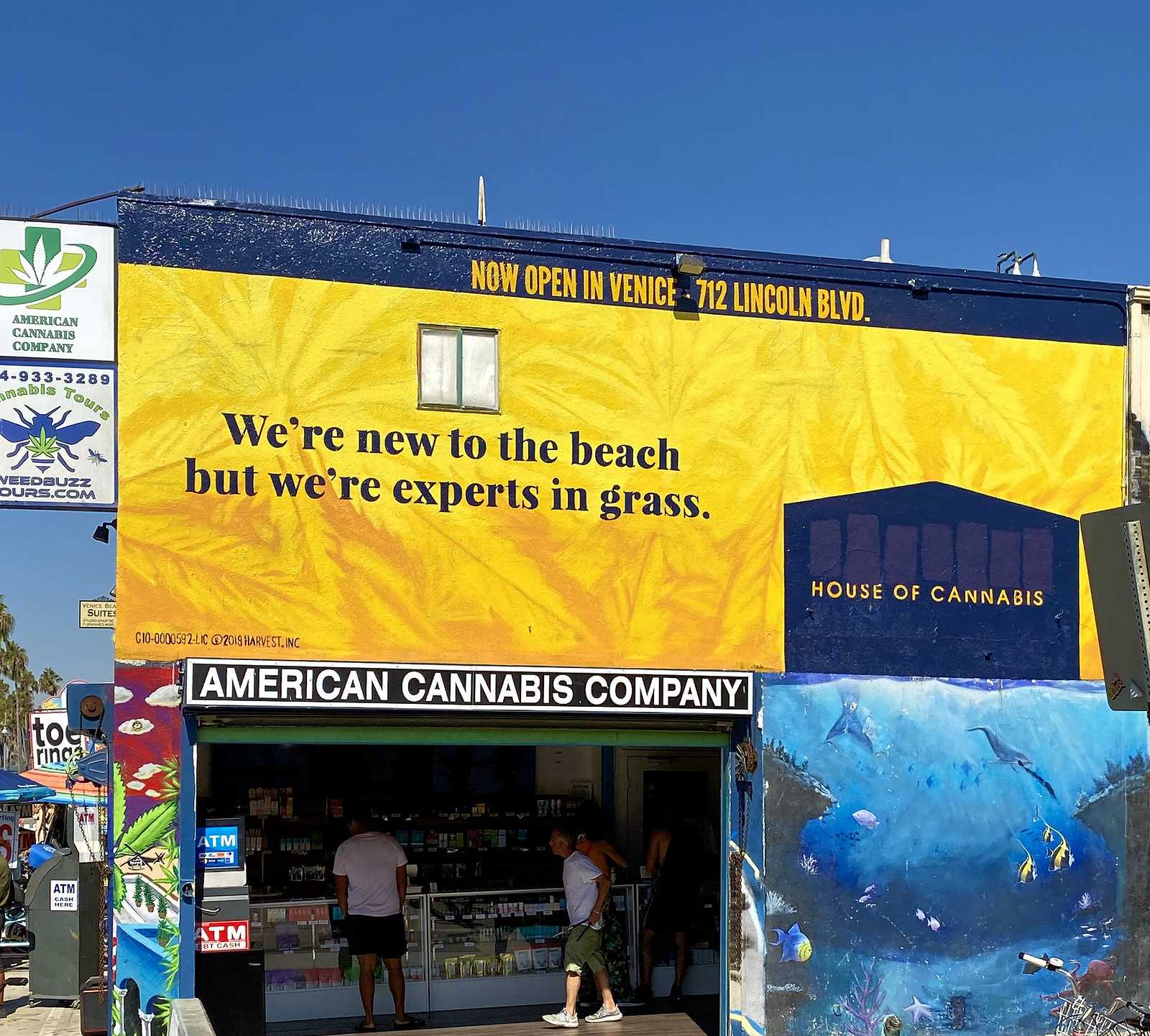The image depicts a two-story building located at 712 Lincoln Boulevard in Venice Beach, California. The ground floor houses the American Cannabis Company, identifiable by a large garage-style entrance and a prominent black and white sign bearing the store’s name. Above the entrance, a large yellow banner reads, "We're new to the beach, but we're experts in grass," with the additional text, "House of Cannabis, now open in Venice." The entrance area is bustling with a couple of people situated in front of a counter displaying various cannabis products. To the left of the main entrance, an ATM is visible near the sidewalk, which features other nearby business signage, including a place offering toe rings and Cannabis Tours. The building is adorned with colorful murals: a vibrant underwater scene with a dolphin and tropical fish on the first story, and a bold yellow background with blue text on the second story. The exterior environment includes some trees and additional street-level elements contributing to the lively atmosphere.